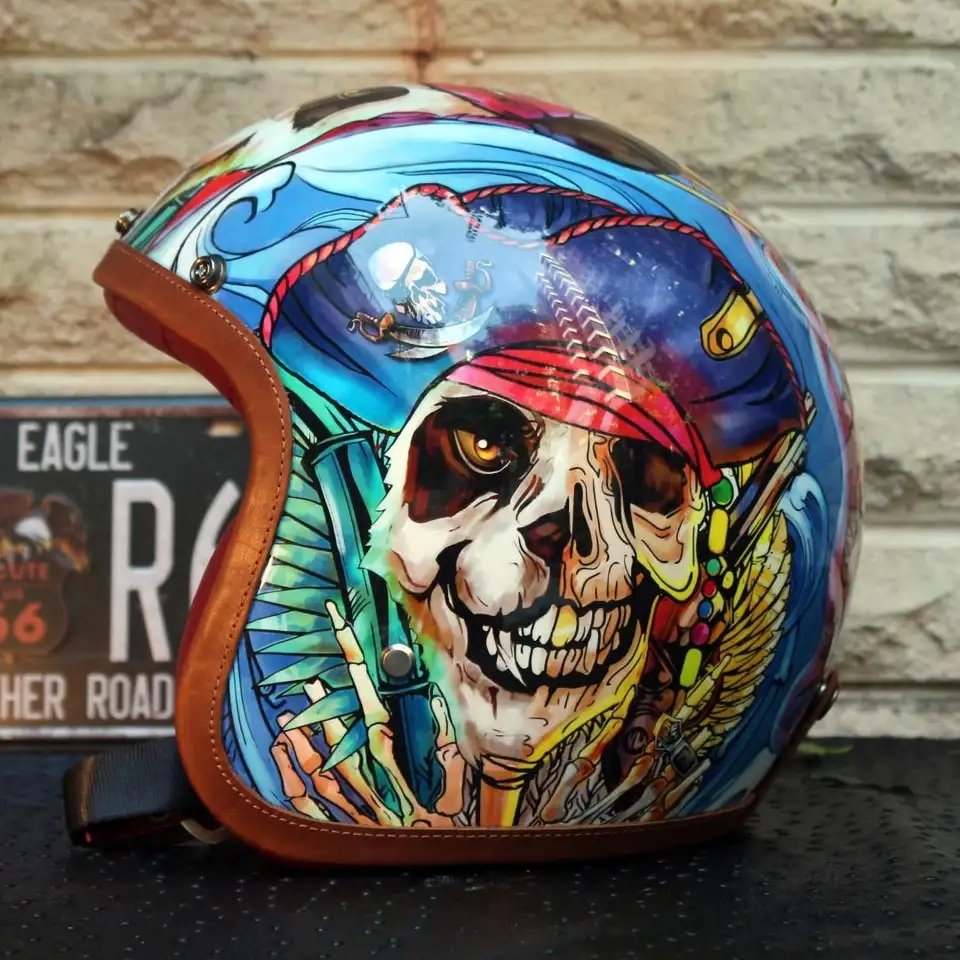The image showcases an intricately designed, visor-less motorcycle helmet resting on a circular black table in front of a light beige and gray brick wall. The helmet features vibrant and detailed artwork predominantly in shades of blue, light blue, dark blue, and aqua. Central to the helmet's design is a striking skull, depicted with a fusion of human and panda characteristics, wearing a red bandana and a blue pirate hat. The skull is accessorized with a golden tooth, and the hand of a skeleton, which appears to be clutching a gun, intertwines with various oceanic and bamboo motifs. Brightly colored elements, such as beads, a yellow feather-like design, and a large blade, accentuate the pirate theme. To the left within the background, a partially visible black license plate with white letters reads "Eagle" and includes fragmented text and half of a Route 66 symbol with an eagle atop it. Overall, this highly detailed composition of the helmet juxtaposes vibrant and macabre elements against the neutral brick background, creating a dynamic visual narrative.